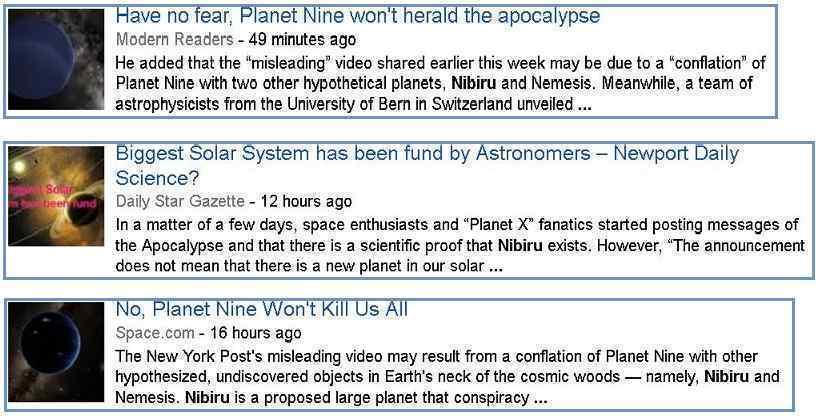This image comprises three distinct boxes, each with a thematic focus on outer space, and is accompanied by varying captions in greenish text against a light green or grayish background.

**First Box:**
This section features an image of a planet in outer space. The heading is in a greenish hue and reads: "Have no fear, Planet Nine won't herald the apocalypse." The attribution line beneath it states "Modern Readers - 49 minutes ago." The accompanying text continues: "The quote misleading end quote video shared earlier this week may be due to a quote conflation end quote of Planet Nine and two of the hypothetical planets, Nemesis. Meanwhile, a team of astrophysicists from the University of Bern in Switzerland unveiled an ellipsis."

**Second Box:**
This section also displays an image related to outer space, with a title in greenish text: "Biggest Solar System has been Discovered by Astronomers." The source is noted as "Newport Daily Science," followed by another source, "Daily Star Gazette - 12 hours ago," with additional text in black: "In a matter of a few days, space enthusiasts and quote Planet X end quote fanatics started posting messages about the apocalypse, claiming there is scientific proof that Nibiru exists. However, the quote announcement end quote does not mean that there is a new planet in our solar system."

**Third Box:**
Again depicting an image of a planet in outer space, this box has a heading in greenish text: "No, Planet Nine won’t kill us all." The source is listed as "Space.com - 16 hours ago," and the body text in black reads: "The New York Post's misleading video may result from a conflation of Planet Nine with other hypothesized undiscovered objects in Earth's vicinity, namely Nibiru and Nemesis. Nibiru is a proposed large planet that conspiracy theorists ..."

Each section provides information on recent astronomical findings and public reactions, emphasizing clarification about the existence and impact of hypothetical celestial bodies like Planet Nine, Nibiru, and Nemesis.